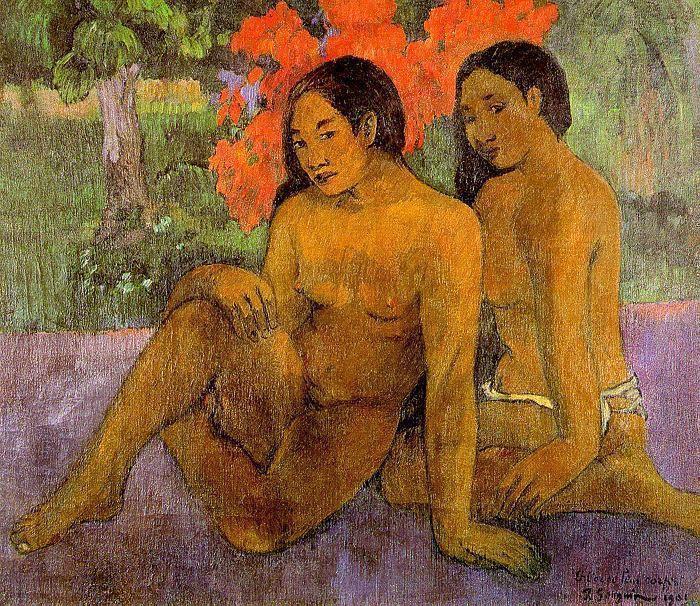This vibrant painting, evocative of Paul Gauguin's signature style, depicts two women with brown skin and long, straight black hair, possibly of Asian or Indian descent. Both are topless, seated on a purple-hued ground that contrasts vividly with the lush greenery behind them. The woman on the right kneels with her back partially towards us, adorned only by a white cloth draped around her waist, gazing over her shoulder. Her position slightly obscures the second woman, who reclines on her left hip with her left leg bent under her right knee. She leans on her left arm while her right hand rests atop her right knee, her hair cascading over her right shoulder. The background features a green landscape punctuated by a large tree on the left, blotches of red suggesting blooming flowers or a bush in the center, and additional foliage completing the scene. The artist's signature, believed to be Paul Gauguin's, is visible in the bottom left corner, dating the piece to 1901. The medium appears to be oil with a touch of pastel effect, lending a rich texture to the composition.